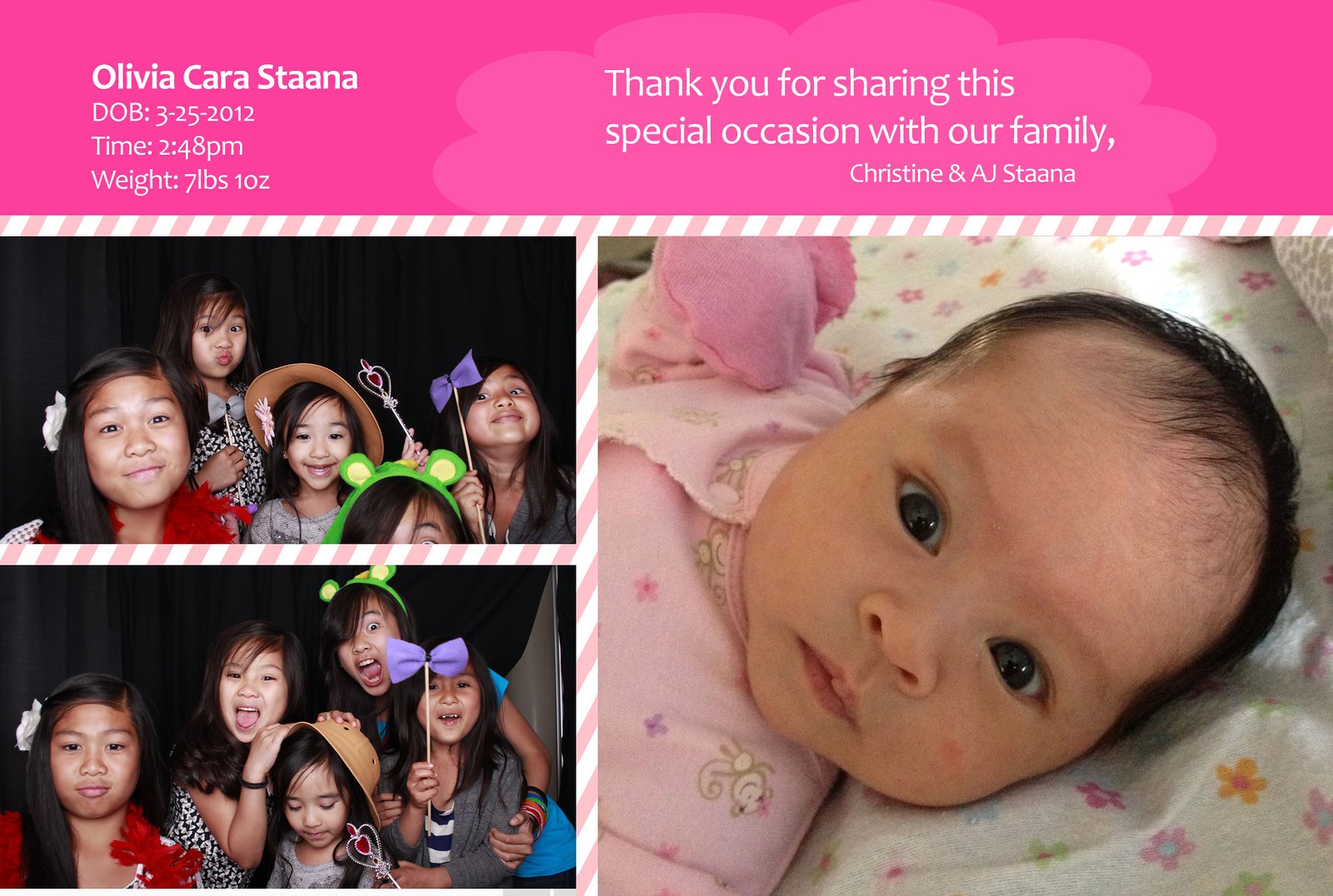The image captures a beautifully designed birth announcement in a landscape orientation, blending color photography with graphic design. At the top of the image, a hot pink horizontal banner with white text details the newborn's information: "Olivia Cara Stana, date of birth 3-25-2012, time 2:48 PM, weight 7 pounds 1 ounce." This is followed by a heartfelt message from the parents: "Thank you for sharing this special occasion with our family, Christine and AJ Stana."

The bottom portion of the image features three photographs. On the bottom right, there's a large square photo of a baby, Olivia, lying in a crib on a white blanket adorned with flowers. Olivia, dressed in a pink onesie, has dark hair and is gazing up at the viewer. To the left of this close-up are two horizontally-aligned photos, stacked one above the other, showcasing five young girls, likely family members. The girls, who have Southeast Asian features, are wearing colorful hats and outfits, and are making playful faces and poses in front of a black curtain backdrop.

The overall color palette of the image includes different shades of pink, white, brown, black, red, green, and purple. The design combines photographic representationalism with graphic elements, set against a pink and white striped candy cane background, creating a joyful and celebratory family picture.